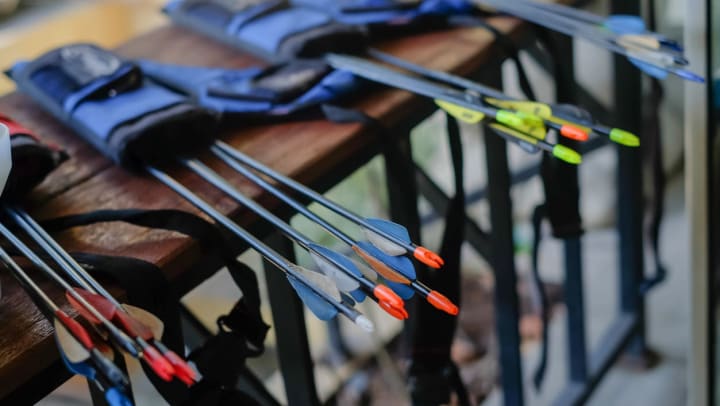The image captures a detailed, focused scene featuring four quivers filled with arrows, lying on a dark brown wooden table with black metal legs. The table stretches from the left-hand side of the frame to the top middle, slightly elevated to the right. Of the four quivers, three are primarily blue and black in color, while one, which is partially cut off by the image's left edge, appears red and black. Each quiver holds about four to six arrows, their dark gray shafts adorned with an array of tail feathers in blue, gray, red, orange, and green hues. The arrows are all angled downward and towards the right. The setting seems likely to be outdoors, possibly at an archery range, indicated by the lack of sharp shadows suggesting an overcast sky. The background and lower part of the table show a slight blur, suggesting a shallow depth of field.